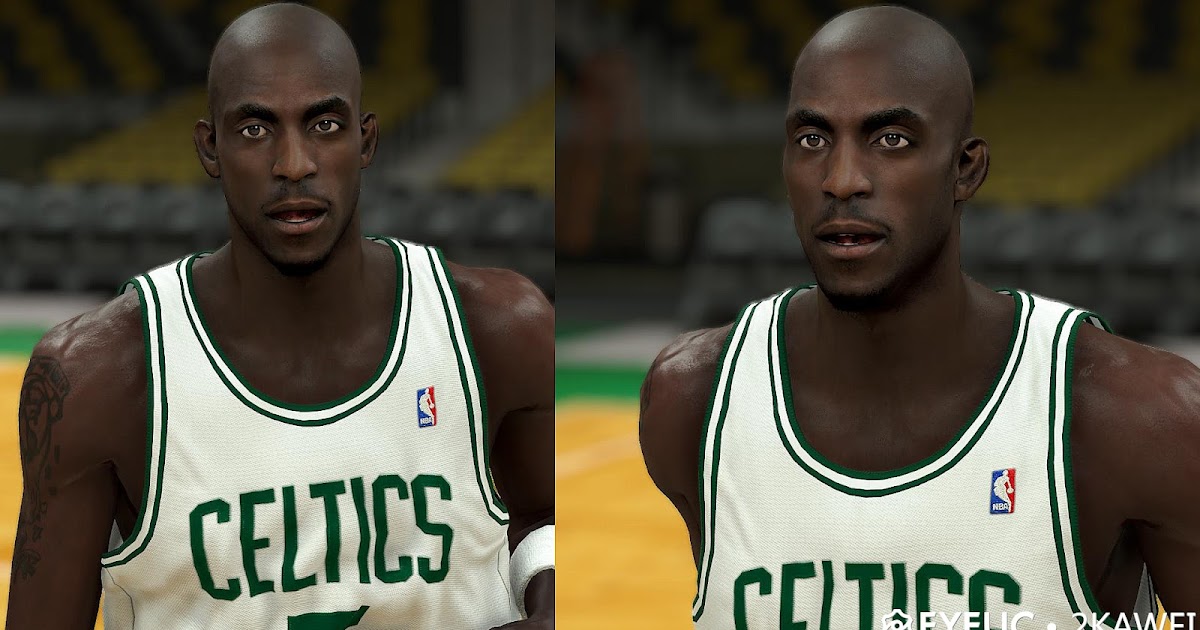This image is a screenshot from a basketball video game, depicting a highly detailed, computer-generated avatar of a player from the Boston Celtics. The scene features two pictures of the same player side by side. The avatar is an athletic Black man with an extremely muscular build. 

In both images, he is wearing a white Celtics jersey adorned with the NBA logo. A noticeable tattoo is visible on his left side, and he sports a sweatband on his arm. His facial features include deeply set brown eyes, well-defined eyebrows, and a mustache. His mouth is slightly open, adding a dynamic expression to his face. 

In the left image, the player is positioned to show both of his ears, while in the right image, he is angled such that only his right ear is visible. His arm posture differs slightly between the two images, with his arm positioned further behind his back in the right image.

The background is void of a crowd, focusing purely on the basketball court, emphasizing the virtual nature of the scene.